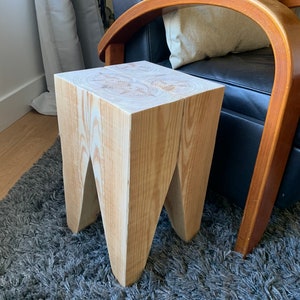The photograph showcases a contemporary styled room featuring a distinctive piece of wooden furniture on a blue shaggy rug. Dominating the image is an end table or nightstand, uniquely designed to resemble a human tooth. This piece is crafted from a single block of wood, with a natural grain finish that is both rustic and designer-like. Its square top, possibly coated with a white resin or paint, contrasts the brown, tooth-like pronged legs that give it a cubist appearance. In the background, a cream-colored baseboard runs along the light wooden panel floor, with gray drapes hanging near the baseboard and wall. Adjacent to the end table is a black vinyl chair with deep-polished wooden armrests, almost semi-circular in shape, and adorned with a white pillow. The cohesive layout of these elements contributes to the room's modern, aesthetic appeal.